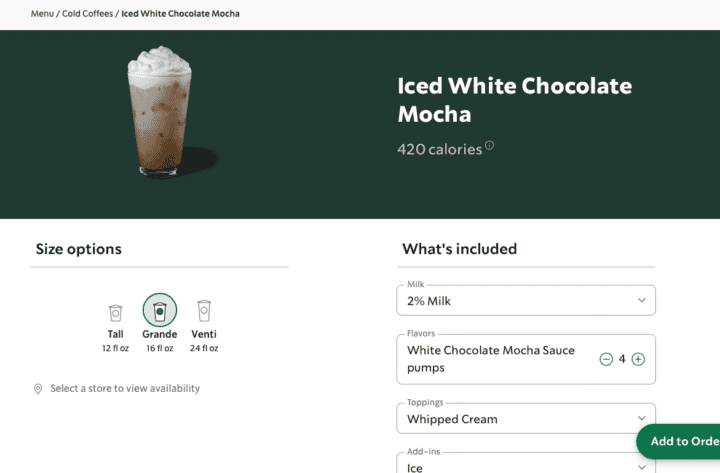This detailed image is of a menu screen featuring a cold coffee option, the "Iced White Chocolate Mocha." At the top of the menu, set against a gray background, is the title "Menu / Cold Coffee / Iced White Chocolate Mocha." The central focus is a large, appetizing photo of the Iced White Chocolate Mocha, showcasing a tall, clear glass filled with chocolate mocha and crowned with a generous amount of whipped cream. This image is placed within a prominent dark green box.

Below the photograph, the text "Iced White Chocolate Mocha" is displayed, followed by the beverage's calorie content, which totals 420 calories. Size options available for selection include 'Tall,' 'Grande,' and 'Venti.' Customers are prompted to select a store to view availability.

There is an interactive map pin icon that can be clicked to show store details. The drink's ingredients are listed, including 2% milk and white chocolate mocha sauce, with customizable options for the number of pumps of sauce. Users can adjust quantities by clicking the plus or minus buttons. Whipped cream is also listed as an ingredient, and a dropdown option lets customers select additional toppings and add-ons, such as extra ice.

At the bottom of the menu, a long green oval button labeled "Add to Order" is present for easy selection, enabling users to modify their order as needed. While the image does not specify the store location, there is an impression of familiarity with the establishment.